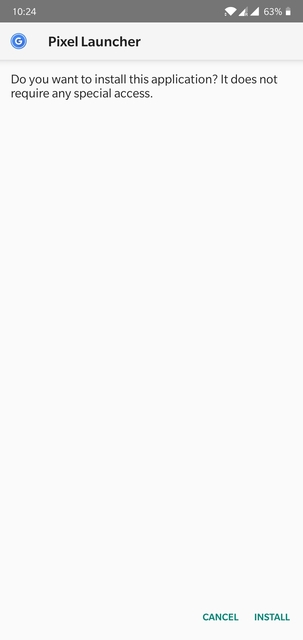The image depicts a smartphone screen showcasing an app installation prompt. Here’s a detailed breakdown of the screen:

At the very top, a status bar is visible. On the far left, the time “10:24” is displayed in white text. Adjacent to it are the Wi-Fi signal strength indicator and two different battery meters. On the far right, the battery life is shown at 63%, marked by a battery emoji.

The status bar has a gray background. Below it, a more prominent header area displays a white "G" encircled in blue, next to which is the text "Pixel Launcher" written in bold, black letters. The header is separated by a faint gray line.

The main content area of the screen is blank and has a light gray background. Toward the center of this area is a straightforward message: "Do you want to install this application? It does not require any special access."

At the bottom right of the screen, there are two turquoise-colored buttons labeled "CANCEL" and "INSTALL." These buttons appear without a border or distinct square outline, blending seamlessly into the UI.

The overall aesthetic is minimalist with a focus on functionality, highlighted by the contrast between the darker top of the screen and the lighter gray of the main content area.